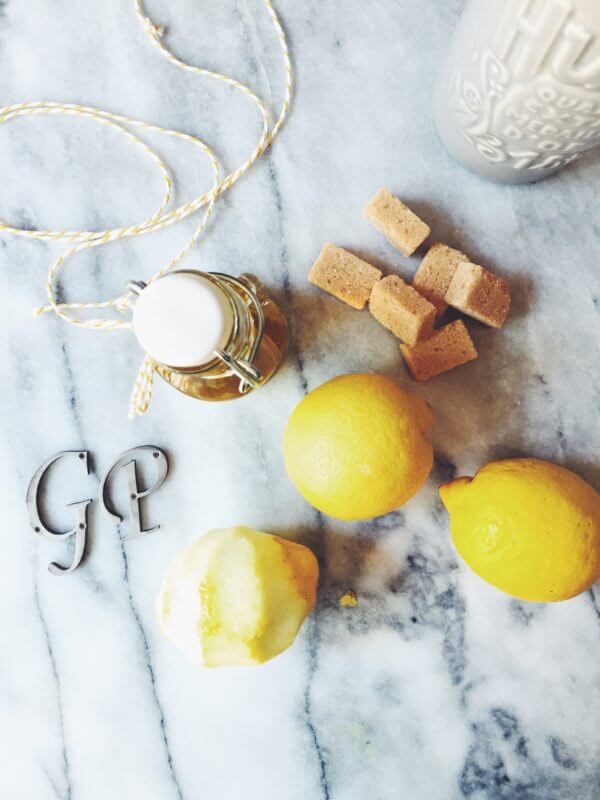The image features a blue and white marble table—primarily white with blue streaks and splotches, especially concentrated in the lower right corner. On this surface, three lemons are arranged, two of which are whole while one is cut in half with its interior facing up. Positioned to the upper left of the lemons are metallic silver letters "GP." Above the letters, a jar with a white metal cap and a metal wire latch is visible, accompanied by a string with white and yellow stripes extending to the upper left corner of the image. In the upper right corner, there is a white cup with engraved text that partially reads "quality extra metal." Below this cup, towards the center of the photo, sit six brown sugar cubes, lying just above the lemons.